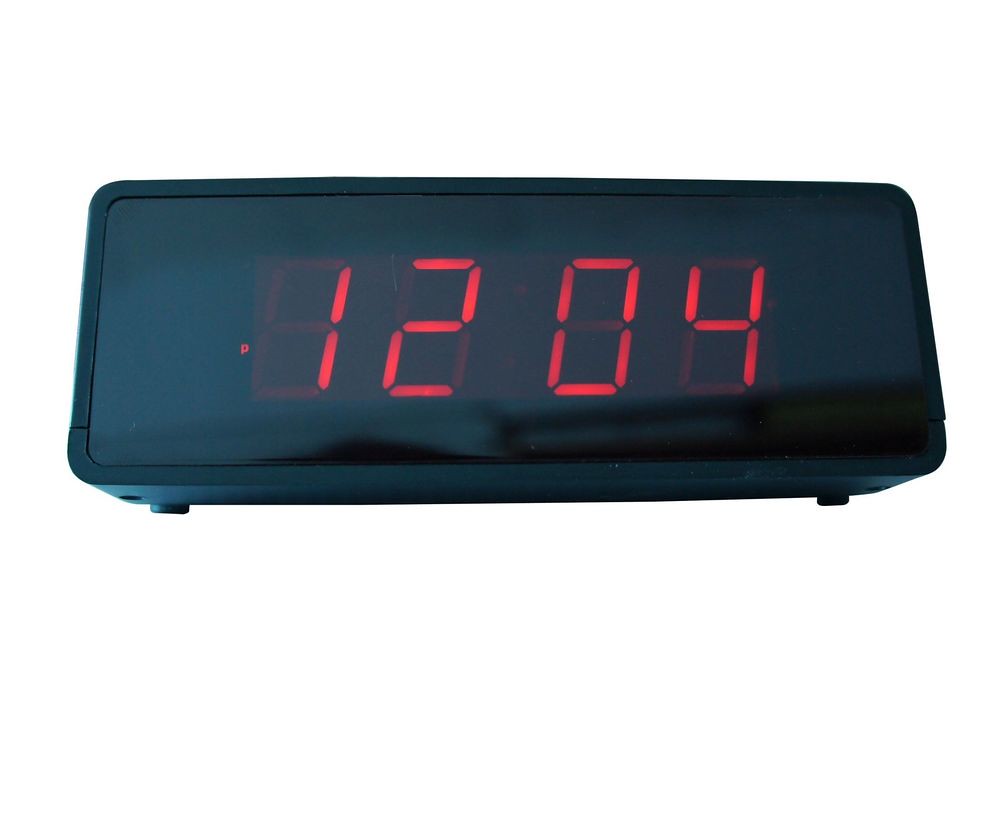The image is a detailed advertisement photograph of a classic digital clock set against a white background. The clock features a black plastic frame with a slightly rectangular shape and rounded edges. Its display shows the time as "12:04" in red digital numbers, along with a small glowing red "P" on the left side, indicating it is 12:04 PM. Notably, there are no separating colons between the hours and minutes on the display. The clock is supported by two round feet visible at the back, adding to its stability. A small round circle, likely a reset button, is situated near the left foot of the clock. The clock's surface has a shiny finish that reflects light, enhancing its sleek appearance.